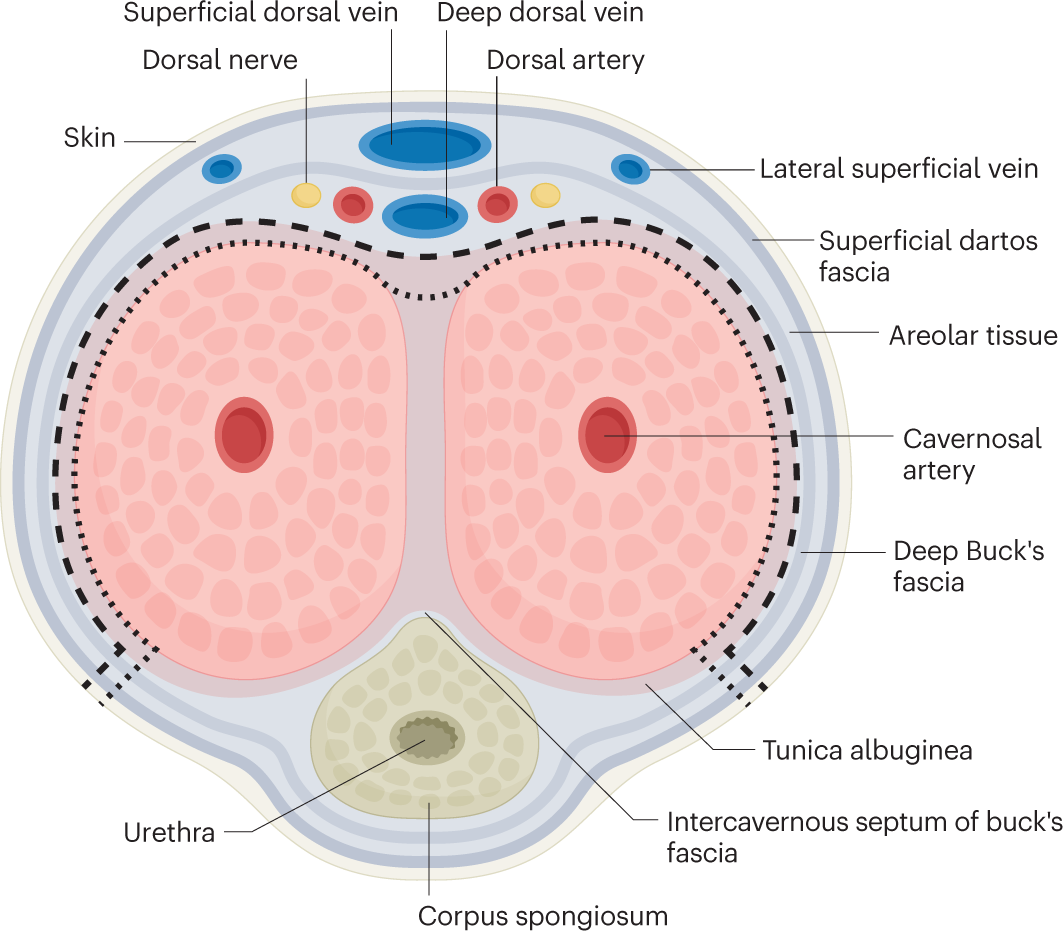This highly detailed and colorful diagram, likely from a textbook, illustrates various parts of human anatomy in a top-down cross-sectional view. The diagram displays an intricate array of components labeled with precise text and indicating lines. Key elements include the skin as the outer boundary, the dorsal nerve, superficial and deep dorsal veins, dorsal artery, and lateral superficial vein. Beneath the surface layers, it showcases the superficial dartose fascia, areolar tissue, cavernosal artery, deep Buck's fascia, tunica albuginea, intercavernous septum of Buck's fascia, corpus spongiosum, and the urethra, depicted in light green. The image, resembling the shape of a skull or head with two prominent round portions tinged in pink and red, uses a vibrant color scheme featuring reds, blues, yellows, and greens to detail the complex vascular structures and tissues, providing a comprehensive visual study for medical understanding.